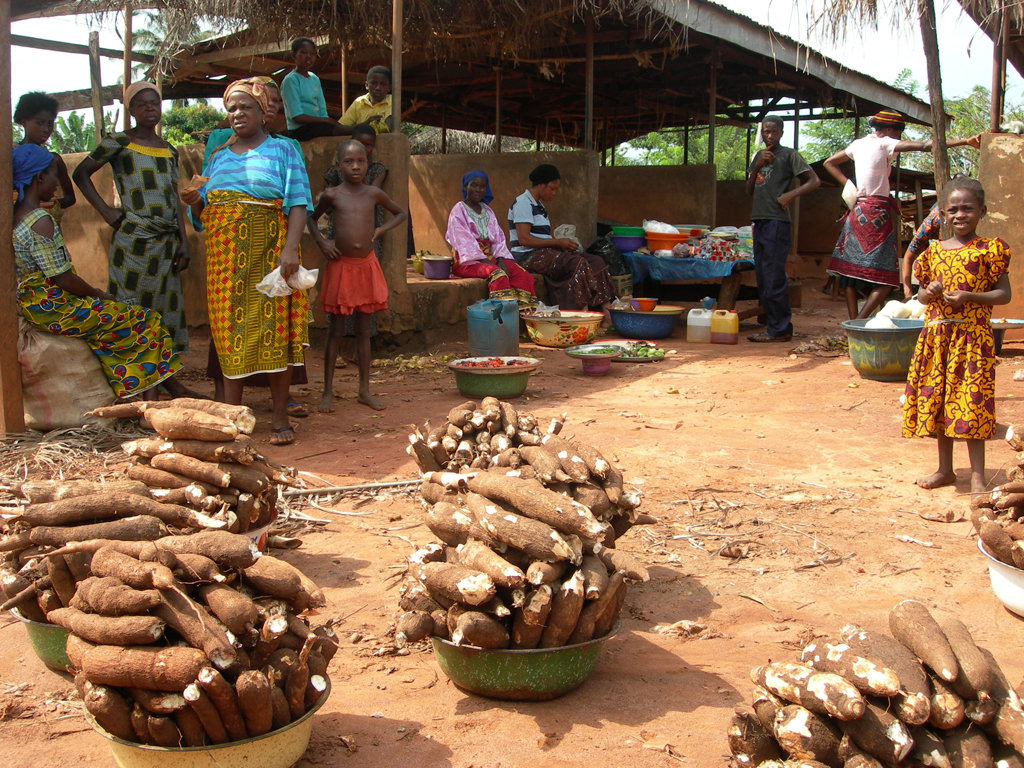In the photograph, an outdoor scene from an African village unfolds, capturing the essence of daily life in a seemingly underprivileged area. The dry, clay-like ground stretches beneath several makeshift structures with incomplete walls but providing necessary shade. In these lean-to setups, people, predominantly women in dresses and aprons, appear to be engaged in activities like cooking or peeling vegetables. Several men and young boys in pants accompany them, signifying a communal effort. Large bowls filled with long, brown root vegetables, reminiscent of yams or sweet potatoes, populate the foreground, heaped high and suggesting a focus on food preparation or harvest. A young girl in a yellow dress stands out among the group, adding a touch of color to the scene. Many individuals look directly at the camera, dressed in native attire, including African waxcloth skirts, enabling a vivid snapshot of their cultural fabric amidst modest surroundings.